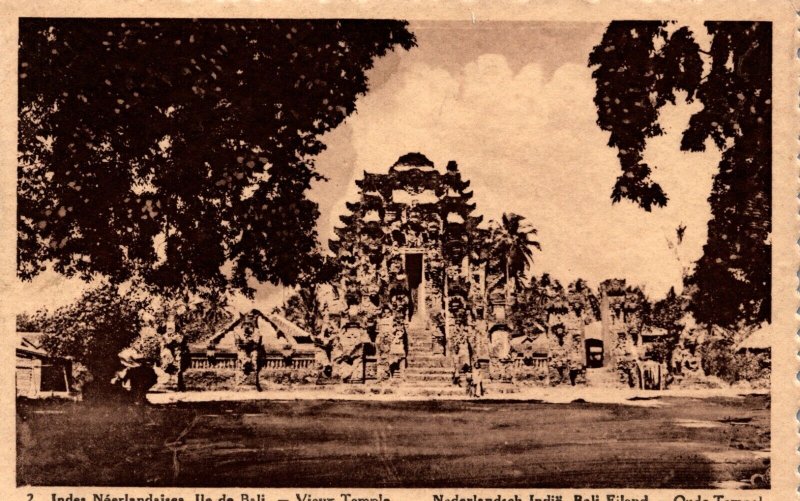The image in question is an extremely yellowed and aged photograph, possibly with a pinkish hue. It has a thin border that shares this coloring, suggesting a combination of factors such as material and age. The photograph depicts a landscape scene featuring what appears to be an ancient South American or tropical temple, possibly Mayan or Incan, with steps leading up to a central door. This main structure is surrounded by several statues, pillars, or totems, which are somewhat indiscernible due to the photo’s blurriness and sepia tones. The bottom 20% of the picture shows water, enhancing the old-world, mystical ambiance. Flanking the temple are very large trees, potentially oaks, with palm trees and other foliage visible towards the top corners. The image is reminiscent of a black and white or sepia postcard or an old newspaper clipping, evidenced by text at the bottom or surrounding the image in a traditional newsprint font. Although the specific text is unreadable, it likely provides context or a description of the scene, hinting at its historical or cultural significance.